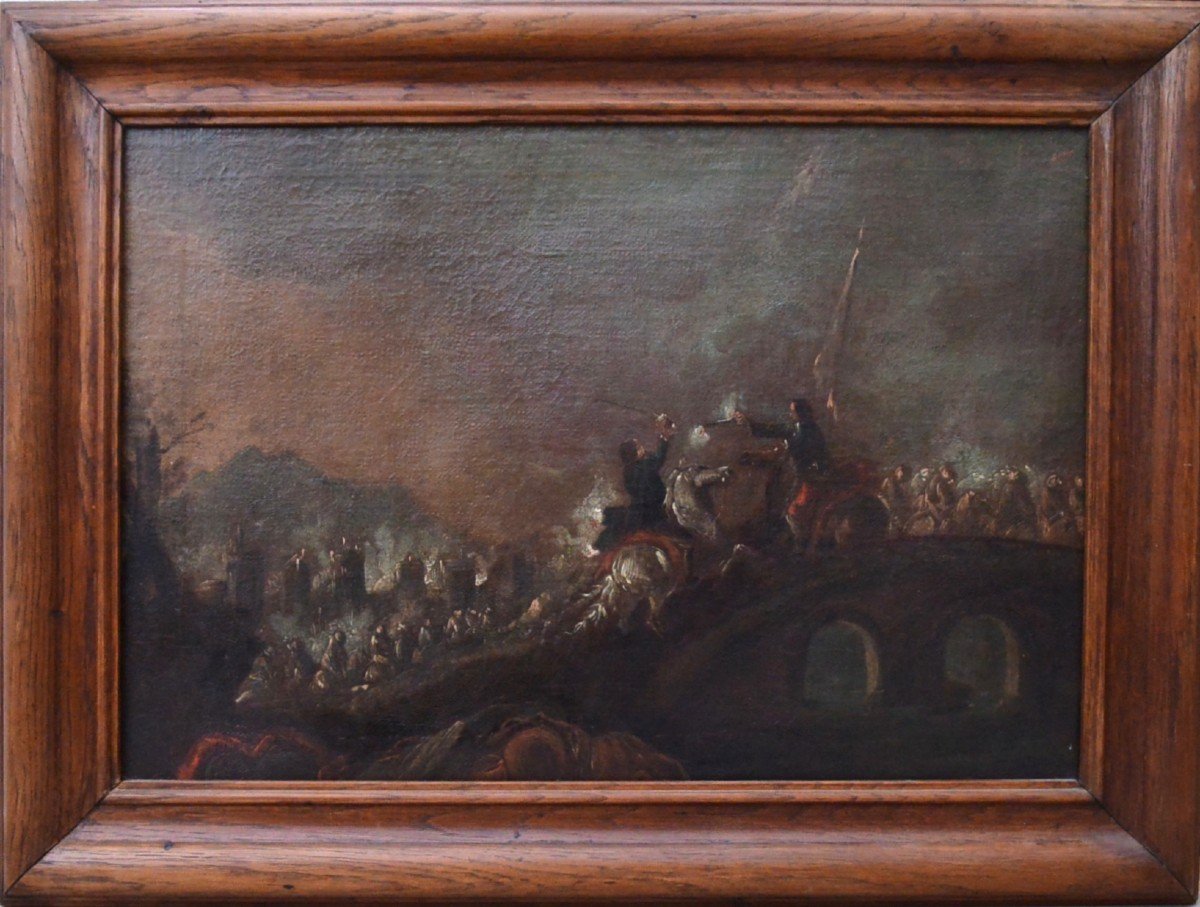This image captures an old, dark-toned painting depicting an intense battle scene framed in dark brown, ridged wood. The painting itself is predominantly shaded in blacks, browns, and grays, with sparse hints of dark orange, particularly near the top left corner. At the center, two men clash on horseback atop a small, curved stone bridge. The man on the left rides a white horse, while the man on the right is mounted on a brown horse. Both men appear to be engaged in combat, with one seemingly drawing a weapon, possibly a sword or a gun. Surrounding them, vague silhouettes and dots suggest more fighters, enveloped in a smoky, clouded landscape with hints of fire. The background of the painting is mostly dark, transitioning from a dark horizon at the bottom to more gray and black tones at the top, enhancing the depiction of a war-torn, chaotic environment.